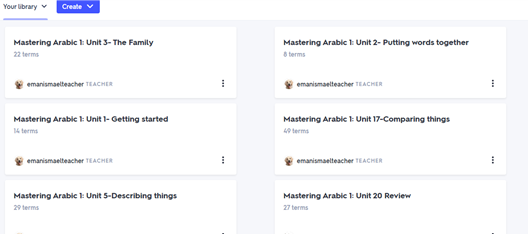The image depicts a web interface displaying a library of educational resources. At the top left corner, there is a small tab labeled "Your Library" with a blue underline and a down arrow beside it. Below this, there's a prominent blue "Create" button. The main content area is divided into two columns, each containing three tabs. 

The tabs in the first column are:
1. **Mastering Arabic 1: Unit 3 - Family** (22 terms) by Iman Ismail Teacher.
2. **Mastering Arabic 1: Unit - Getting Started** (14 terms) by Iman Ismail Teacher.
3. **Mastering Arabic 1: Unit 5 - Describing Things** by Iman Ismail Teacher.

The second column features:
1. **Mastering Arabic 1: Unit 2 - Putting Words Together** by Iman Ismail Teacher.
2. **Mastering Arabic 1: Unit 17 - Comparing Things** by Iman Ismail Teacher.
3. **Mastering Arabic 1: Unit 20 - Review** by Iman Ismail Teacher.

All these elements are set against a gray background, providing a clear and organized view of the available study units within the library.